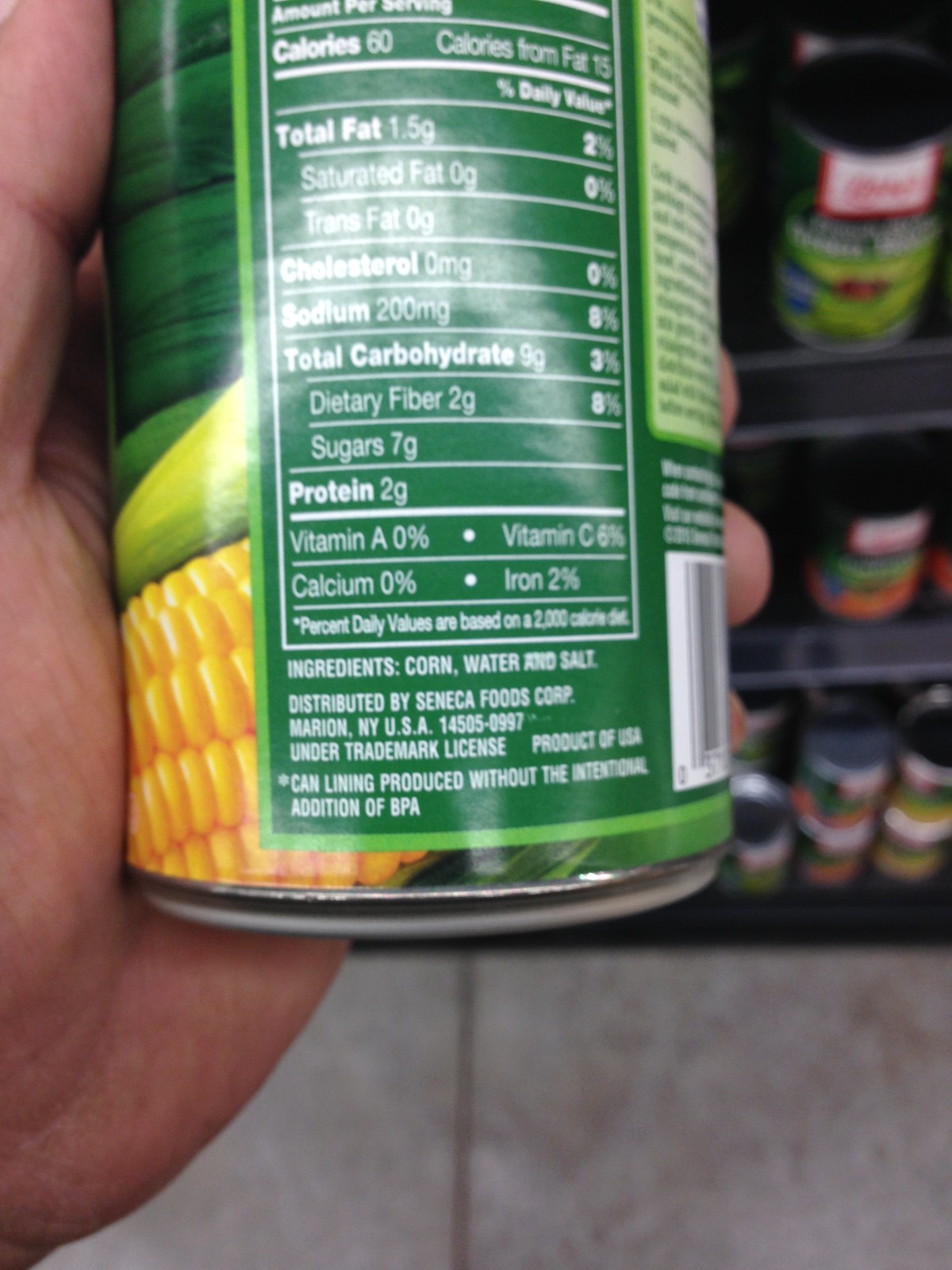In a brightly lit supermarket, a close-up color photograph captures a green can of corn held in the left hand of a shopper. The hand, with its thumb and part of the fingers visible, showcases the back of the can prominently featuring the nutritional facts label. Detailed information includes 60 calories per serving, 1.5 grams of total fat (2% DV), with 0 grams of saturated and trans fats, 0 milligrams of cholesterol, and 200 milligrams of sodium (8% DV). The total carbohydrates are listed as 9 grams (3% DV), with 2 grams of dietary fiber (8% DV), 7 grams of sugars, and 2 grams of protein. Vitamins and minerals are also noted, including 0% vitamin A, 6% vitamin C, 0% calcium, and 2% iron. The ingredients list states corn, water, and salt. The background reveals shelves lined with various canned vegetables, identifiable by their red and white tags, possibly Libby's, stacked in an orderly manner, adding to the bustling atmosphere of the store.